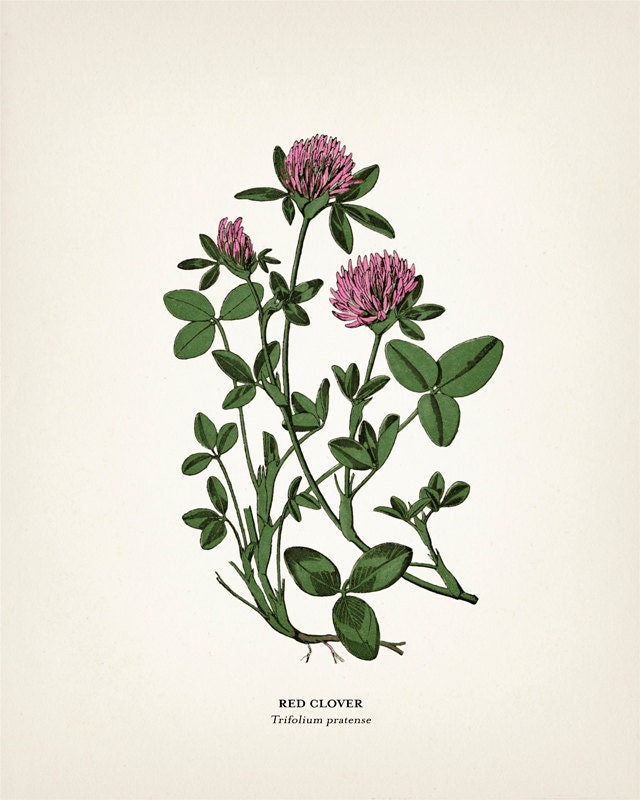In this meticulously detailed illustration, we see an artistic and scientific depiction of a Red Clover (Trifolium pratense), centered against an ivory white background with a hint of pale lilac. The botanical print features an array of dark green stems that extend from the bottom, where short roots are visible, pulling out from an imaginary ground. Surrounding the stems are numerous gray-green three-leafed bunches, each leaf marked by a darker green stripe from tip to base. The focal point of the illustration is the clover's blossoms, depicted with medium to deep purple, thistle-like petals that form round clusters. One of the flowers is seen as a budding shoot with petals moving upward, while two others are in full bloom, showcasing their spiky, detailed petals with subtle gray shadows. The illustration is captioned at the bottom, “Red Clover, Trifolium pratense,” emphasizing its scientific and artistic significance.